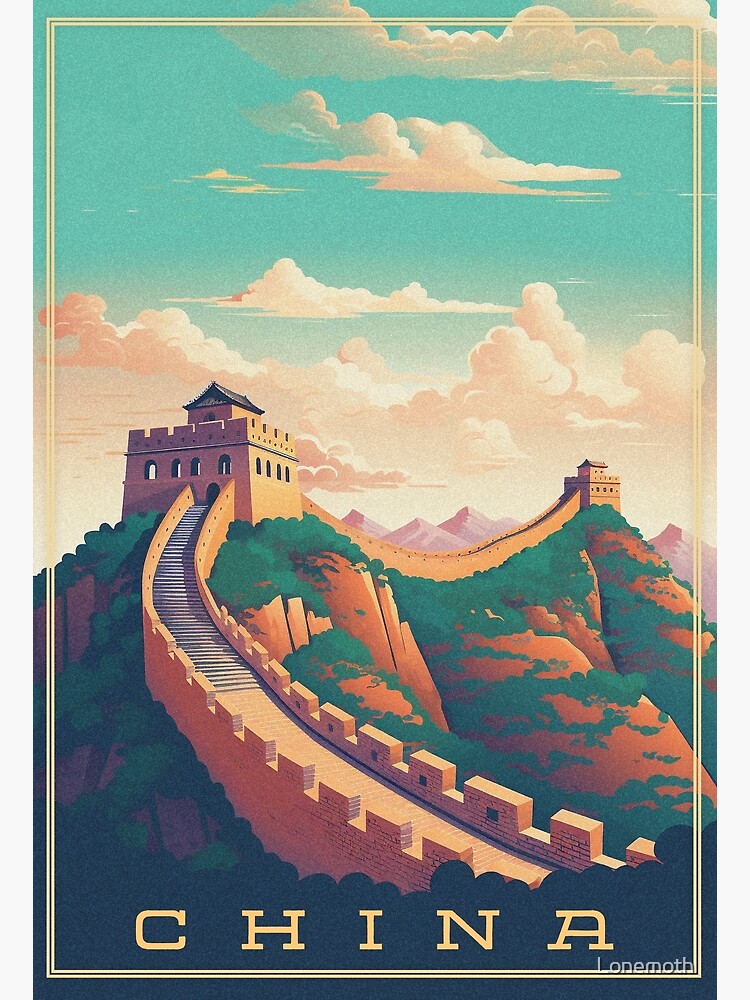This is an intricately illustrated postcard depicting a picturesque scene of the Great Wall of China. The central focal point of the image is a light brown structure, reminiscent of a block house with windows. This building is connected by an extensive pathway, not quite a staircase, featuring black lines that give it a stepped appearance, weaving up the green, grassy hillside. Above this structure, the sky is a striking sea-foam blue, interspersed with clouds, creating a serene backdrop against the rugged mountains in the distance. At the bottom of the postcard, the word "China" is boldly inscribed in a light beige or yellowish hue. The entire image is encased in a yellowish border, contributing to its postcard-like charm. The colors are mainly vivid greens from the grass, a yellowish tint of the Great Wall, and the bluish-green of the sky, lending a vibrant, almost painted quality to the scenery.